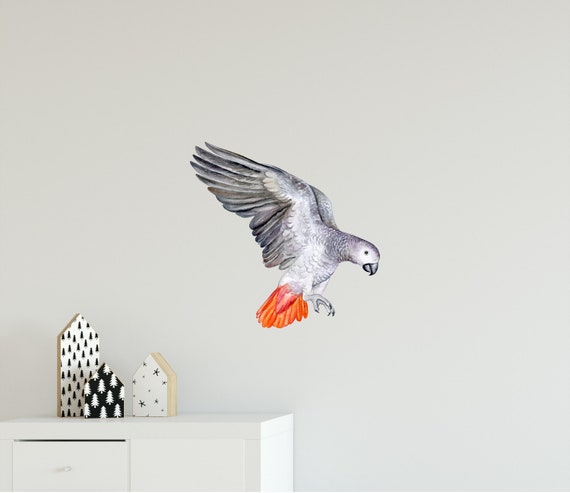The photograph features a striking African gray parrot in mid-flight, prominently placed at the center of the frame. Captured in an indoor setting, the bird is soaring against an off-white wall, its wings outstretched with feet extended as if poised to pounce. The parrot's plumage is predominantly gray, marked by darker wing feathers streaked with black, and a vivid tail showcasing hues of orange and red. The bird's white chest and distinctive white mask around its small black eyes, along with its black beak, are clearly visible in its profile view as it faces the right side of the room.

In the lower left-hand corner of the image, part of a chest of drawers is visible. This white dresser has a slightly open drawer and is adorned with decorative items on top. These decorations include stylized house-shaped figures in black and white, each adorned with patterns featuring stars, trees, and dots. Two of the figures resemble fir trees, while the third features multicolored stars. The parrot, comparable in size to a black crow, creates a dynamic and detailed focal point against the minimalist indoor background.